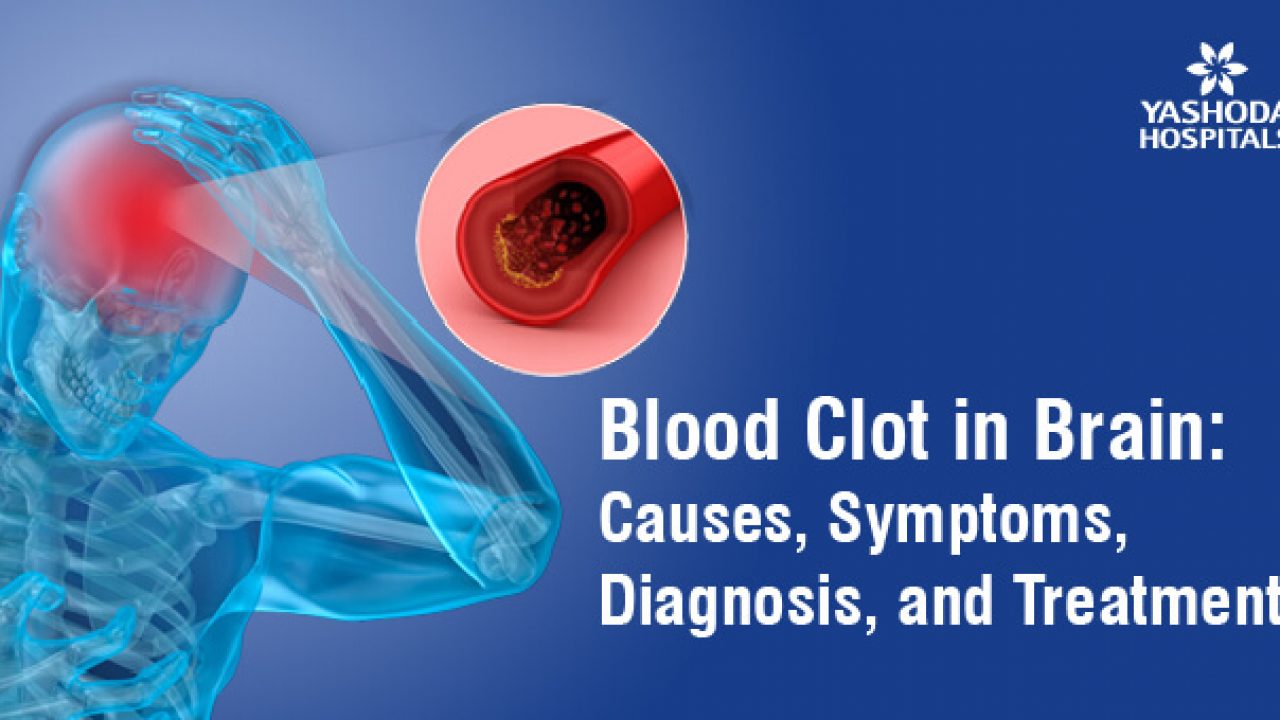The image is an advertisement flyer for Yeshoda Hospitals, featuring a detailed and striking visual to convey its message. The background transitions from dark blue to lighter blue in the upper left corner. In the top right corner, there's a star-shaped or flower-shaped white logo, slightly cropped, with the text "Yeshoda Hospitals" (though the 'A' in 'Yeshoda' and 'S' in 'Hospitals' are barely visible). On the left side, there's a computer-generated image of a semi-transparent blue human figure, showcasing a skeletal structure with a red-highlighted area on the brain, indicative of pain or a medical issue. A close-up circular inset details a red artery with an apparent obstruction inside, illustrating a blood clot. Below, bold white text reads: "Blood clot in brain: Causes, Symptoms, Diagnosis, and Treatment."